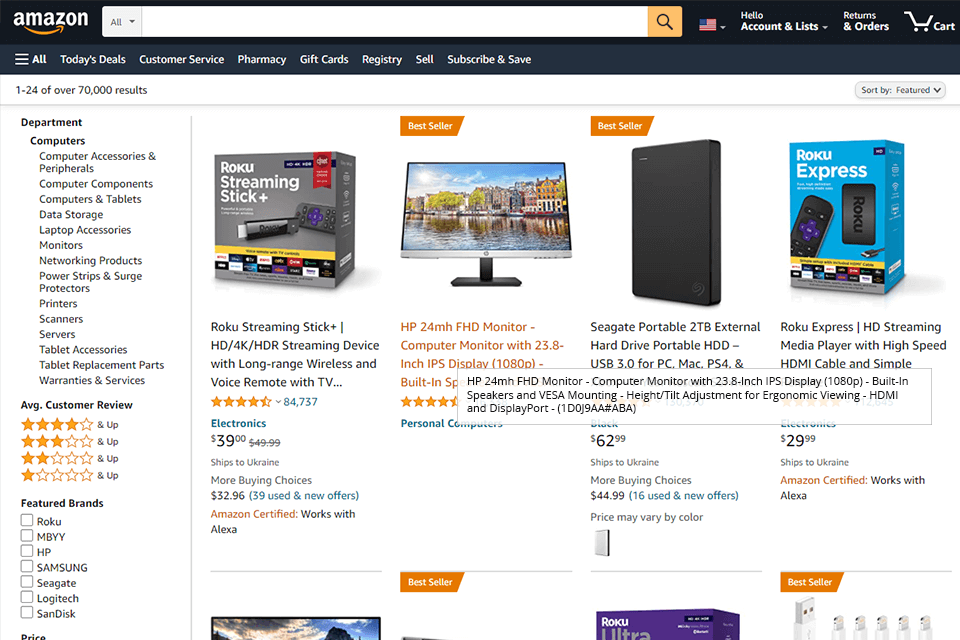The Amazon web page features a sleek black header adorned with the Amazon logo situated on the far left. Centrally located is a search box equipped with a dropdown menu that is currently set to "All," allowing users to narrow their search to specific categories. Adjacent to the search box, users can find an American flag with an arrow, enabling the selection of different languages. To the right, "Hello, Accounts & Lists" serves as a dropdown menu, alongside quick access to "Returns & Orders," and an icon of an empty shopping cart.

The left navigation bar is tailored to the current browsing context, displaying a statement: "1 to 24 of over 70,000 results," despite the search box being empty. Users can refine their search by choosing departments; under "Computers," subcategories like "Computer Accessories & Peripherals," "Computer Components," "Computers & Tablets," "Data Storage," "Laptop Accessories," "Monitors," "Networking Products," "Power Strips & Surge Protectors," "Printers," "Scanners," "Servers," "Tablet Accessories," "Tablet Replacement Parts," and "Warranties & Services" are available. Additional filters include "Average Customer Review" and "Featured Brands."

The main content area showcases a variety of products, including a Roku Streaming Stick, a 24-inch IPS display monitor, a 2TB external hard drive from Seagate, and a Roku Express. A pop-up window displaying product information about the monitor mirrors the details found on its label.